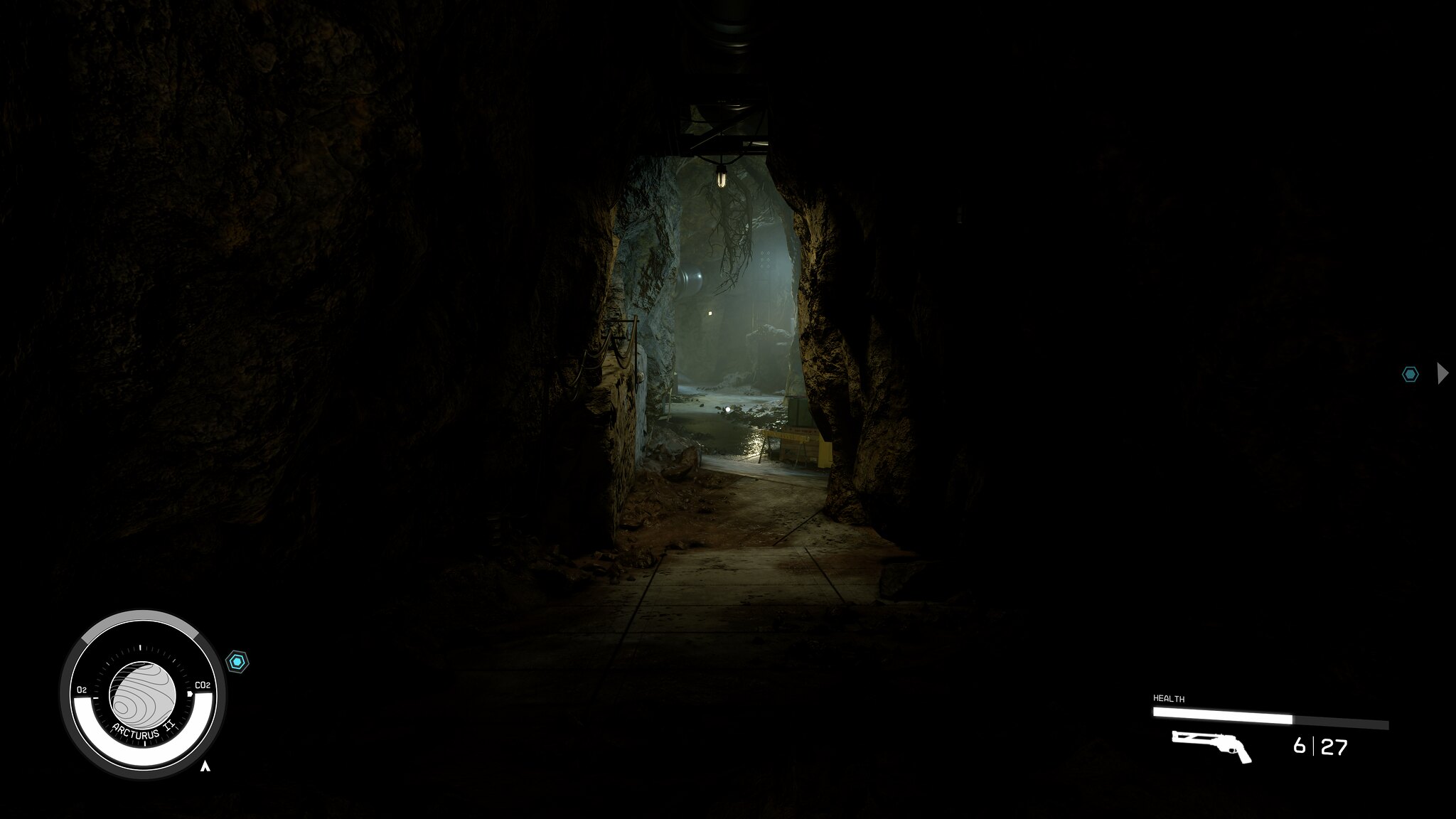In this screenshot from a video game, the viewer gets an immersive, first-person perspective as the player peers into a dimly lit cave hallway. The image is rectangular, with the top and bottom sides being longer than the left and right sides. The cave's entrance dominates the center, showing a complex network of multiple routes that extend from the ceiling. Deep shadows cloak both the left and right sections of the image, rendering them almost entirely black and adding to the eerie atmosphere of the scene.

In the bottom left corner of the screen, part of the game's HUD (Heads-Up Display) is visible, featuring a gray circle with a planet at the center, intricately detailed with gray lines. Beneath the planet icon, there's a white semicircle. On the bottom right, the HUD shows an outline of a gun symbol, next to the numbers "6" and "27," separated by a line—likely indicating ammunition count. Above the gun icon, a white line, half-filled with remaining health or shield status, is partially gray, further contributing to the game's immersive interface.